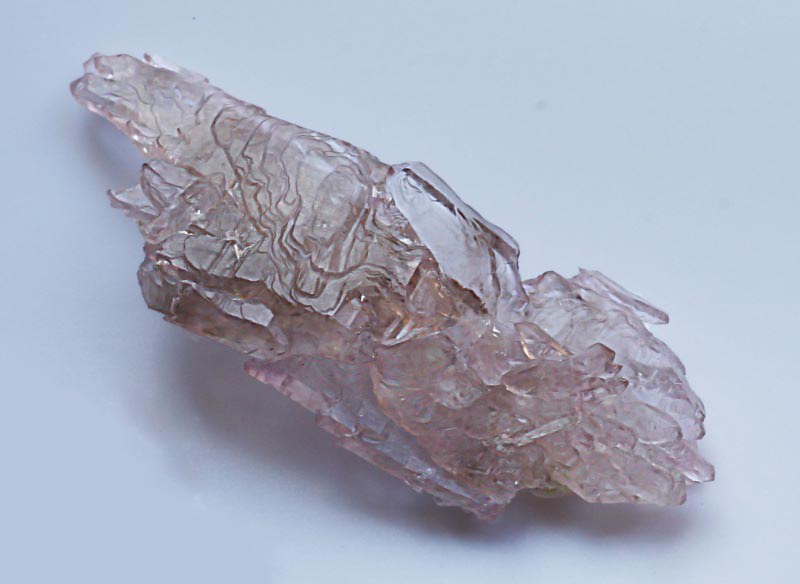The photograph features a striking mineral specimen, possibly representing a clear to pinkish crystal, lying on a light blue surface that could be paper or a desk. The crystal has a distinctly irregular, jagged texture with notable changes in elevation, making it appear wild and unrefined. It stretches from the top left corner to the bottom right in a roughly cylindrical shape with the left and right edges tapering off thinner than the central part. The top side of the crystal extends a bit longer than the bottom. The crystal exhibits a smoky clear appearance with hints of a glass-like or melted glass quality, which might suggest it could be beryl, fluorite, or quartz. The overall shape has been likened to a hand pointing upwards and to the left, with three erect fingers and a bumpy, ridged form resembling curled thumb and pinky. The upper portions of the image are clearer, while the lower right section transitions to a blurrier appearance. The intricate details highlight numerous sharp, jagged sections akin to small geological formations, contributing to the crystal's raw and unorganized aesthetic.